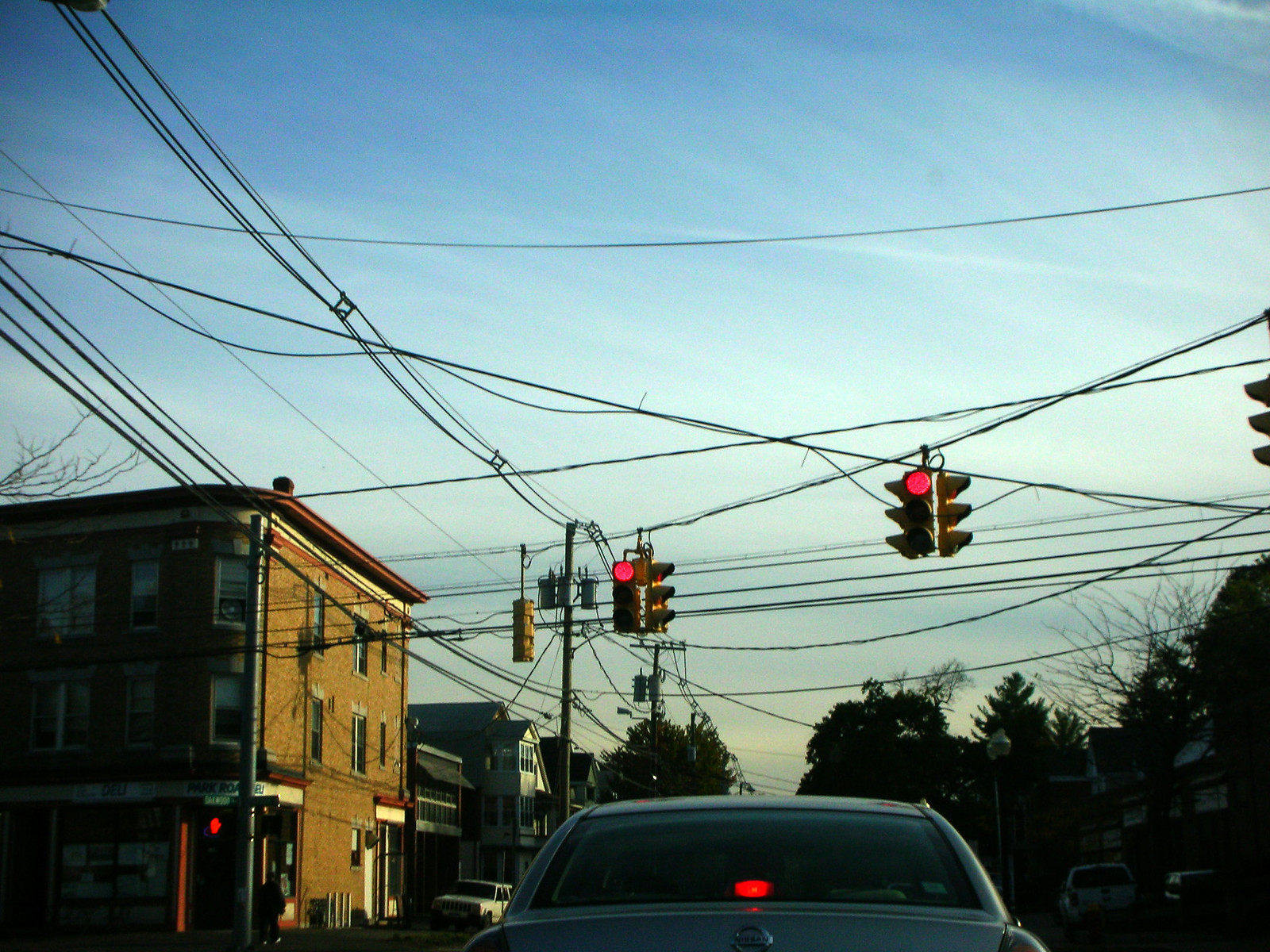This photograph captures a driver's perspective from inside a car, looking through the windshield. In the foreground, a silver-colored Nissan is directly ahead, with its taillight illuminated and visible through the rear window. The scene is set at a busy intersection, indicated by two prominently displayed traffic lights in the distance, both showing red. These traffic lights are distinct with their vertical, three-tiered yellow metal frames, suggesting multiple connected signals possibly governing a multi-stop crossing, though the full extent is not entirely visible in the image. The upper portion of the photograph is crisscrossed with numerous power lines, adding a web-like texture against the backdrop. The sky above is a clear blue, peppered with thin, wispy white clouds. To the left, a tan brick building stands, adding an urban touch to the scene. The overall image portrays a moment paused at an intersection, framed by the typical elements of city infrastructure.